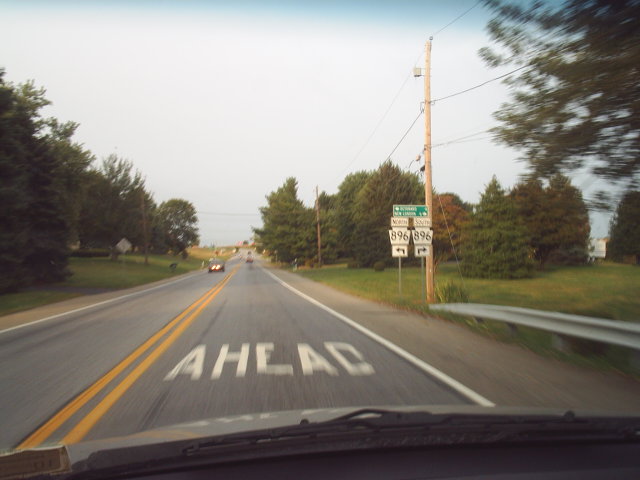The photo captures a long, straight, two-lane road viewed from inside a car, framed by the windshield. The road is marked with double yellow lines in the center and single white lines on its edges. The word "AHEAD" is prominently painted in white block letters on the asphalt. In the opposite lane, a red car with its lights on approaches, while another car is visible in the distance in the same lane we're traveling. The right side of the road features a silver guardrail that slopes downward, adjacent to a wooden telephone pole and a cluster of road signs. Among these signs are dual white signs displaying the number "896" with directional arrows, and a green sign perched on top, though the text on it is unreadable due to the distance. The scenery on both sides of the road is lush with greenery; bushy, evergreen trees dominate the right side alongside patches of grass, indicating a rural setting. The left side also features large trees and grassy areas that resemble front yards. The sky overhead is blue, adding to the peaceful ambiance of the rural road.